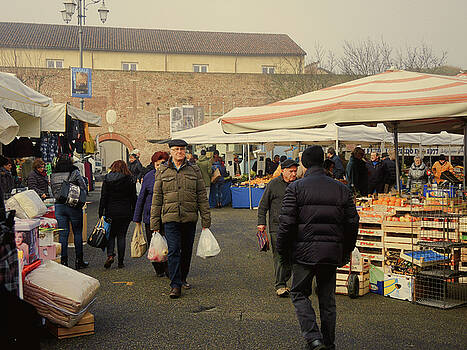A daytime photograph captures a bustling outdoor market in a small European town during cold, cloudy weather. The market, set against the backdrop of two prominent buildings—one an old brick structure and the other a yellow building with a brown shingle roof—features street-side stalls and kiosks under makeshift tents and tan umbrellas. Multiple lampposts adorned with banners line the street. Vendors are selling an assortment of goods including fruits, groceries, and clothes. One prominent stall on the right, recognized by its pale reddish pink striped umbrella, is filled with wooden crates overflowing with apples. Another nearby stall appears to be selling oranges. Shoppers of all ages, both male and female, walk through the market, many bundled in coats and carrying bags filled with their purchases. In a specific scene, a man holding two semi-transparent white bags filled with fruits stands out. The market atmosphere is lively despite only around 20 people being present, with visitors either inspecting goods or engaging with vendors.